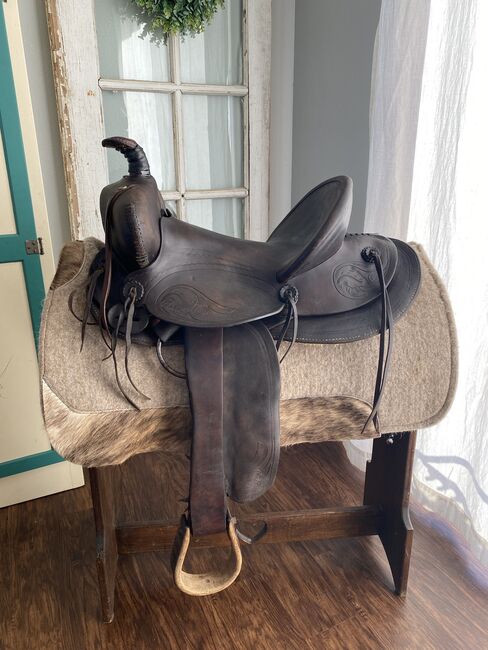The image presents a dark brown leather saddle perched on a wooden saddle stand in a room with distinct details. The stand resembles the body and legs of a horse with a curved, possibly fur-padded gray top, and sturdy wooden legs that are dark brown and connected by a horizontal bar. This saddle, displaying a significant lighter brown buckle and thick straps with stirrups, is oriented with the front on the left and the rear on the right. The scene includes a well-worn, brown wooden floor and is set against a backdrop featuring an old window on the left, framed by an aged wooden trim and covered by a thin, white curtain through which daylight filters. To the right of the saddle, there's a white door adorned with green borders and rectangular glass panes, showing signs of wear with paint starting to strip, and part of a wreath hanging at its top.